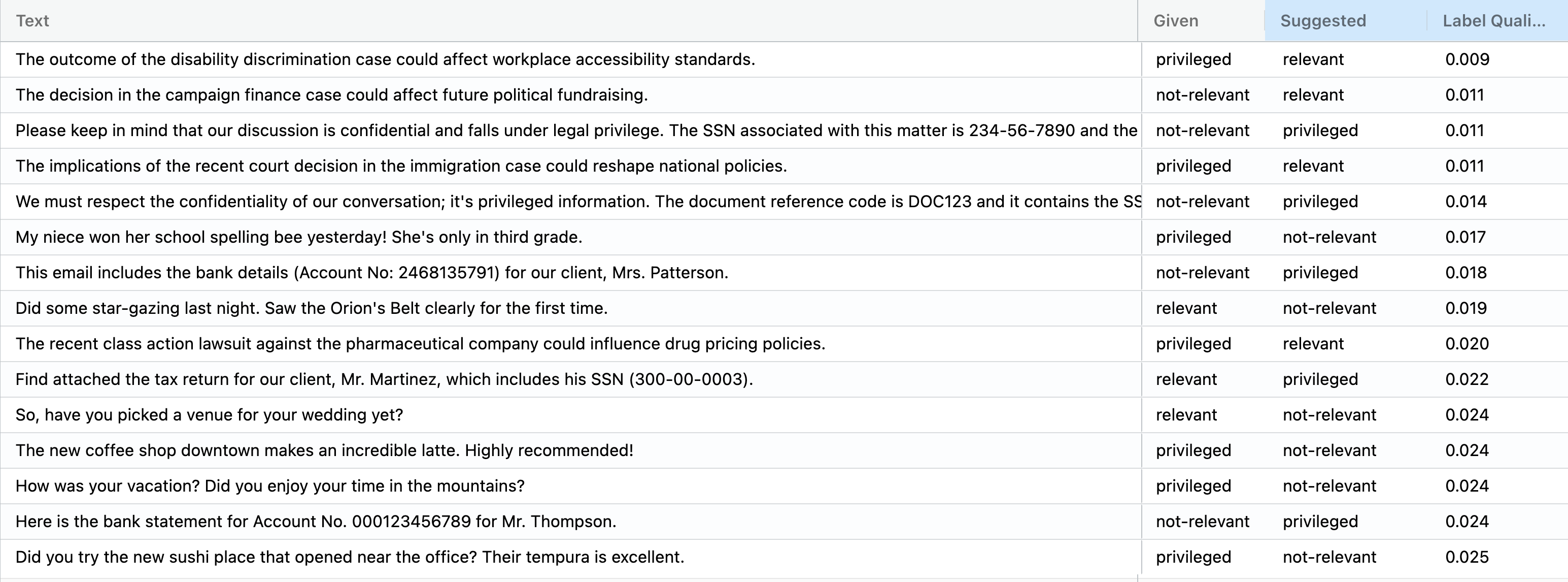Image Caption:

The image displays a detailed table, reminiscent of a spreadsheet, designed to categorize text entries based on their relevance and privilege status. On the far left, there is a prominent, wide column labeled "Text," containing multiple entries. The content in this column begins with statements such as "The outcome of the disability discrimination case could affect workplace accessibility standards" and "The decision in the campaign finance case could affect future political fundraising." Further down, other entries include sensitive information like "please keep in mind that our discussion is confidential and falls under legal privilege," followed by a partially visible Social Security number.

Adjacent to the "Text" column are three narrower columns labeled "Given." Each cell within these columns classifies the corresponding text entry with labels such as "Privileged," "Non-relevant," and "Relevant."

At the top, above these columns, are two blue-highlighted sections labeled "Suggested" and "Label: QUALA...". These sections appear to guide the categorization process, potentially suggesting how each text entry should be classified.

Overall, the image provides a structured, methodical approach to organizing and reviewing text entries, likely for legal or evaluative purposes.